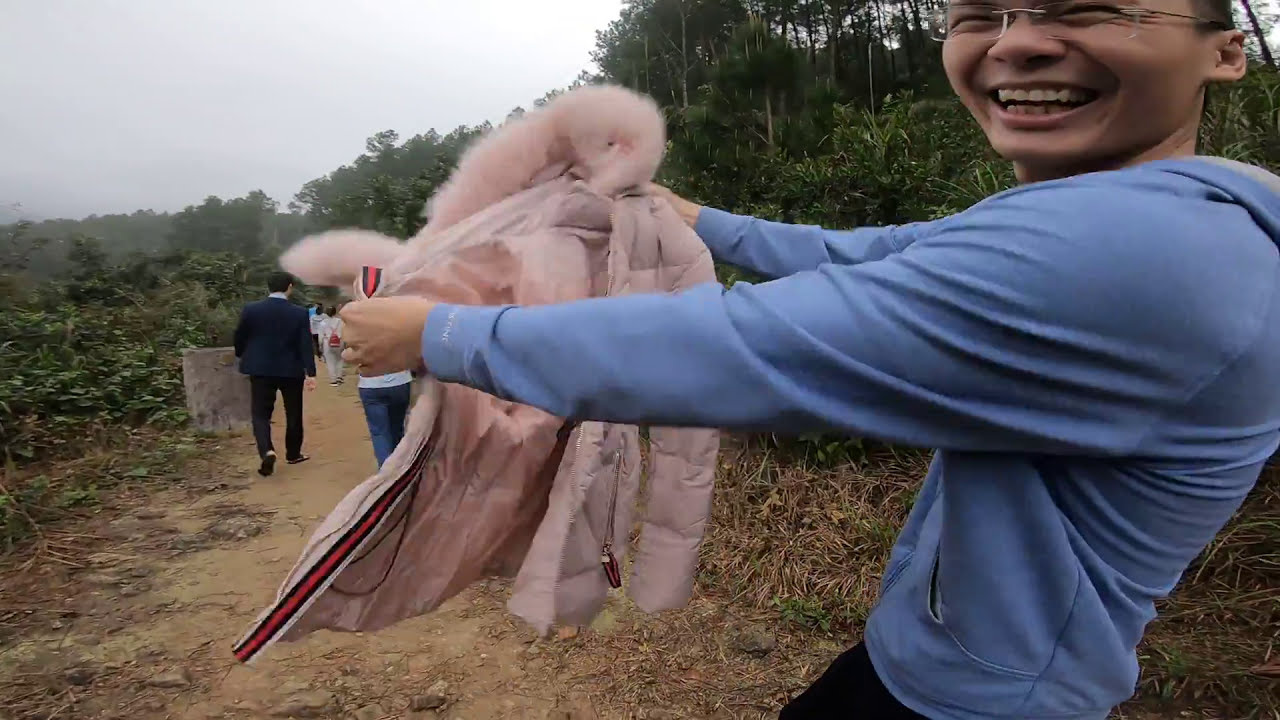In this vibrant outdoor photograph, a person stands prominently on the right side of the image, taking up a significant portion of the frame. They are dressed in a blue hoodie-type shirt and black pants, wearing glasses, and radiating a big smile. The person, appearing joyful, holds a small pink jacket with both hands outstretched. The jacket features a puffy section around the neck and some red striping, suggesting it is not their own. To the left of the person, a dirt path extends from the bottom left towards the center of the image, occupied by several people walking, possibly hiking. Surrounding the scene are lush trees and plants, indicating a natural, wooded setting. The sky peeks through in the upper left corner, adding to the daytime atmosphere. The colors in the image are diverse, ranging from shades of green to gray, brown, red, black, pink, blue, and silver, enhancing the lively and cheerful ambiance of the photograph.